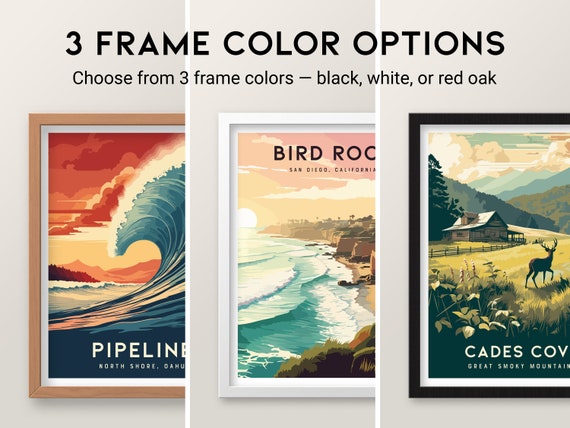The image advertises three frame color options: black, white, or red oak. At the top, bold black text reads, "Three Frame Color Options," and below it, in smaller black text, "Choose from three frame colors: black, white, or red oak." The image showcases three distinct paintings in corresponding frames. On the left, a vibrant painting of a wave against a red sky, titled "Pipeline, North Shore, Oahu," is enclosed in a red oak frame. The central image, featuring a beach scene with cliffs and a pink sunrise, is titled "Bird Rock, San Diego, California," and is set in a white frame. The rightmost image, "Cades Cove, Great Smoky Mountains," depicts a deer near an old farmhouse amidst a mountainous backdrop, encapsulated in a black frame. These segmented images highlight the different frame color options available, each enhancing the respective artwork's aesthetic.